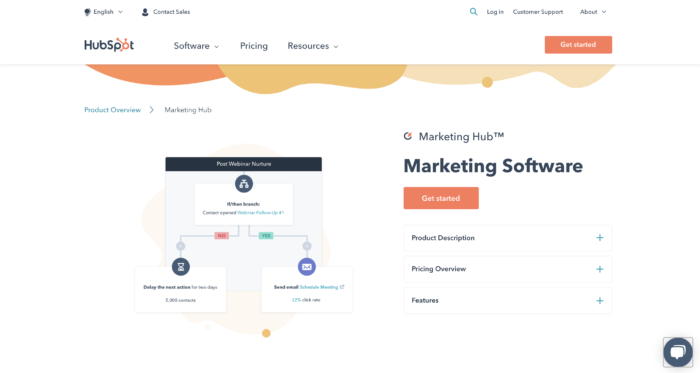This image is a meticulously captured screenshot from HubSpot, a renowned and established content marketing platform. The top header of the interface boasts a clean, white background, prominently displaying the HubSpot name and logo on the left. "HubSpot" is written in a distinctive dark gray font: a capital 'H' followed by lowercase 'ub', a capital 'S', and then lowercase 'pot'. Notably, the 'o' is rendered in orange, featuring three emanating lines with tiny dots at the endpoints—one line pointing straight up, one to the left, and the third pointing to the lower left. The remaining letters return to dark gray, crafting a cohesive and recognizable logo.

To the right of the logo, the navigation menu reads "Software," "Pricing," and "Resources," each accompanied by a small inverted triangle indicating the presence of a dropdown menu. Further to the right, an eye-catching orange rectangle invites users with the white text "Get Started."

Beneath this top navigation area, there is an abstract, decorative element consisting of scalloped designs in gradients of orange, tan, and peach. This artistic detail segues into the primary content area of the page, which also features a white background.

The main section showcases the text "Marketing Hub™" in large, dark gray font, signifying trademark status. Just below, in bold, the text "Marketing Software" is presented, followed by another prominent orange rectangle button labeled "Get Started" in white text. Under this call-to-action button, a series of expandable sections is listed in gray font: "Product Description" with a plus sign to its right for more details, "Pricing Overview" similarly accompanied by a plus sign, and "Features" also expandable via a plus sign.

On the left side of the main content area, a small rectangular diagram with a black border can be seen. This diagram appears to be a visual representation, featuring a central box connected to a box on the left and another on the right, though the specific details and text within the diagram are too small to discern clearly.